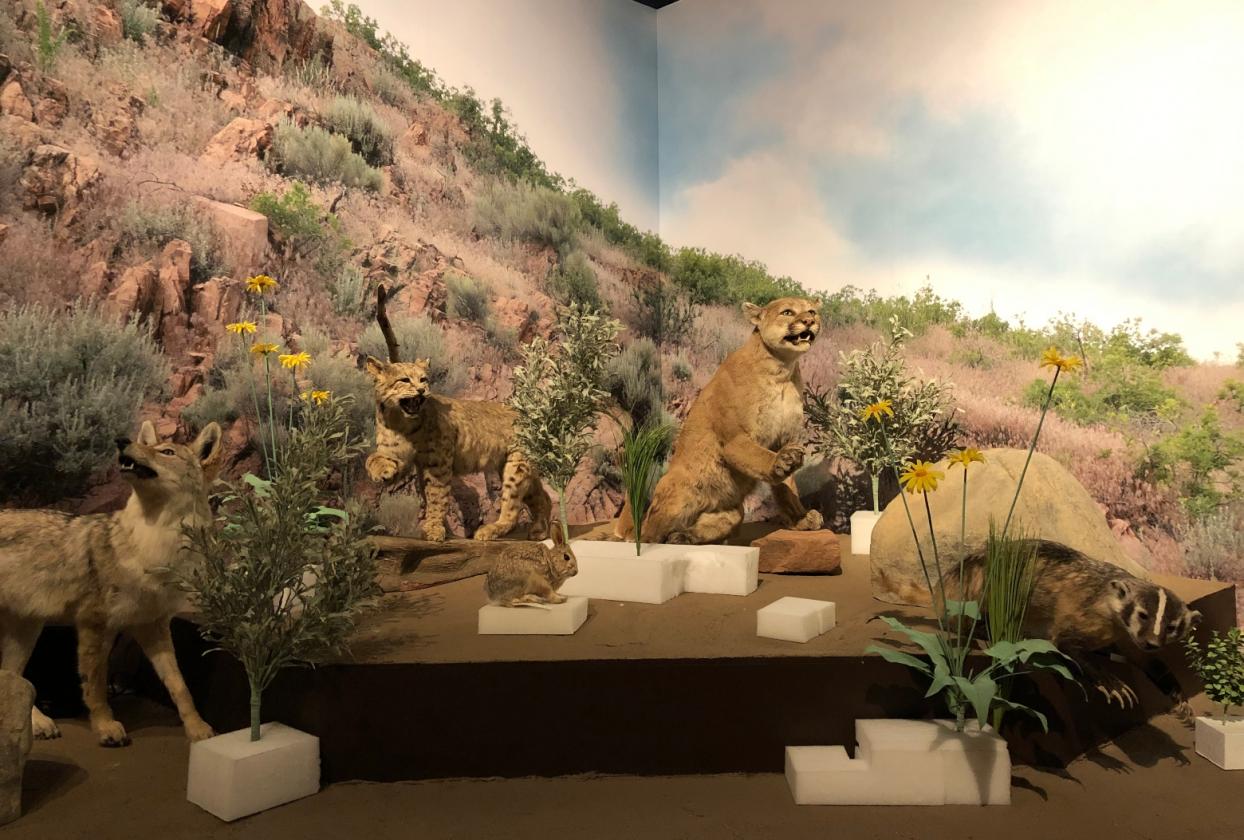This detailed photograph captures an indoor museum exhibit featuring meticulously crafted replicas of various wild animals, all posed to mimic their natural behaviors. Centered around a vivid background poster of a savanna-like landscape with mountainous regions, dry shrubbery, rocks, short grasses, and sparse bushes, the scene is enhanced by an array of plant props in the foreground to evoke a wild habitat setting.

The exhibit showcases an impressive collection of life-sized, taxidermically preserved animals, each carefully placed to tell a visual story. Among the featured animals are a cougar and a bobcat spotted prominently amidst the display, alongside other felines such as a lynx characterized by its distinct fur designs. There is also a coyote or jackal, a common hare, and a wolverine, often associated with forest environments but intriguingly included in this dry landscape scene, adding a layer of geographical curiosity.

This visually compelling exhibit artfully blends educational elements with detailed artistry to present a realistic and immersive experience of wildlife in a savanna-like ecosystem.